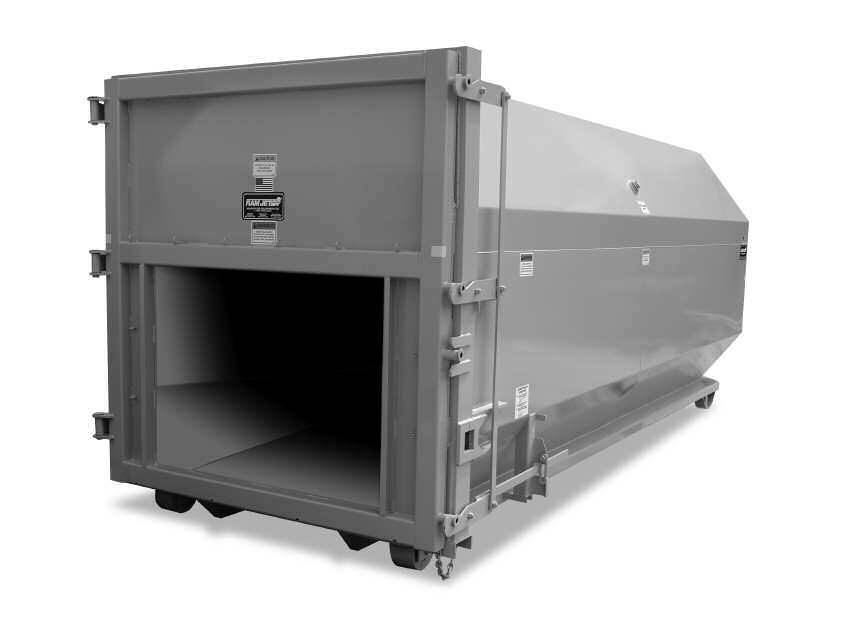The image depicts a heavy-duty, industrial device with an octagon-shaped cylindrical body, appearing somewhat like a large storage tank or possibly a trash compactor. It is primarily a silvery-gray color and rests on four wheels, one at each corner, making it mobile. The device is placed against a white background. On the front of the device, there is a prominent opening or entry point, which might serve as the compartment for depositing materials. This entry space reveals a dark interior. The machine features an intricate locking mechanism and is adorned with several tags, including a visible American flag sticker, indicating it might be made in the USA. Additionally, there are several warning stickers, although the specific text on them is not legible.